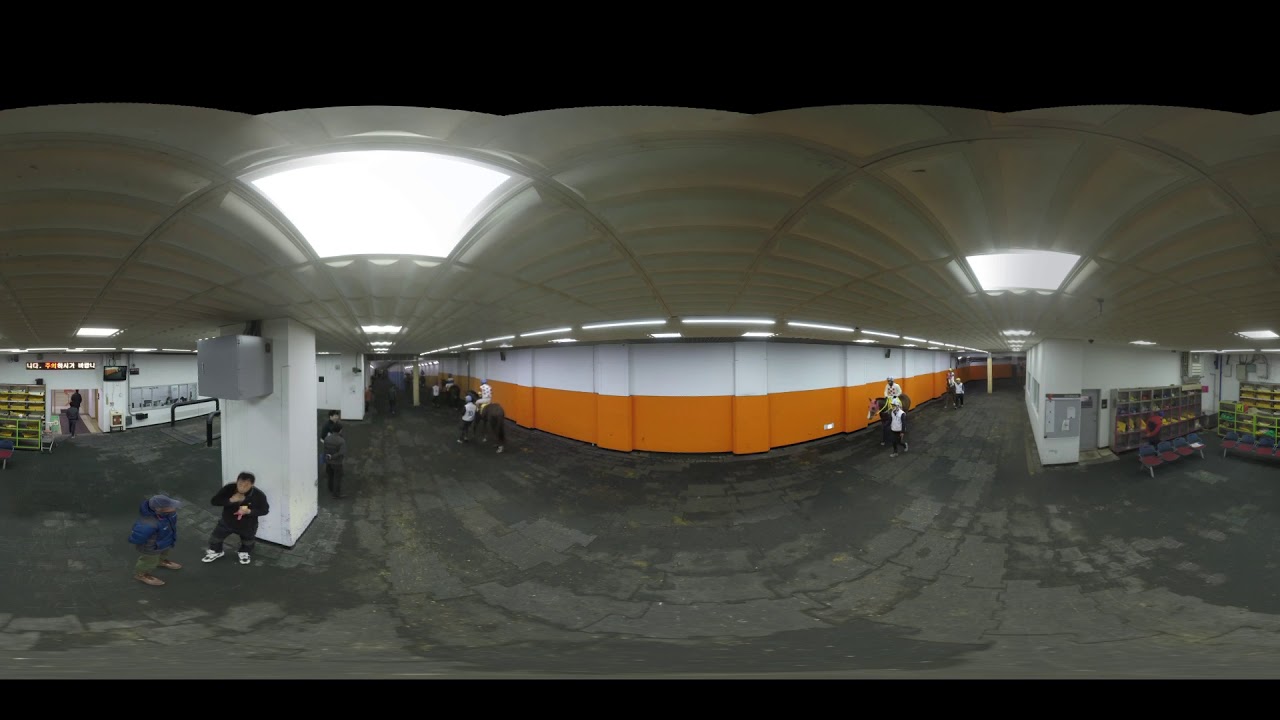This fisheye, panoramic image captures an indoor scene that resembles a large underground corridor, potentially within a subway station, arena, or warehouse. The predominant flooring is made of black-gray asphalt, and the environment is well-lit by a grid of fluorescent lights on the ceiling. Various industrial fixtures, such as shelves and breaker panels, are visible, along with a series of bins on the right and a doorway on the left. The walls are mostly white with sections of bright orange near the bottom. In addition to the eclectic mix of people walking about, several individuals are seen riding horses, suggesting that this area could serve jockeys and their horses either as a stable or a prep area before an event. The image is framed by thin black borders at the top and bottom, adding to the encapsulated, 360-degree viewpoint which slightly distorts the scene's linear features. This unique perspective highlights the bustling activity and multifaceted utility of the space, merging the mundane with the unexpected.